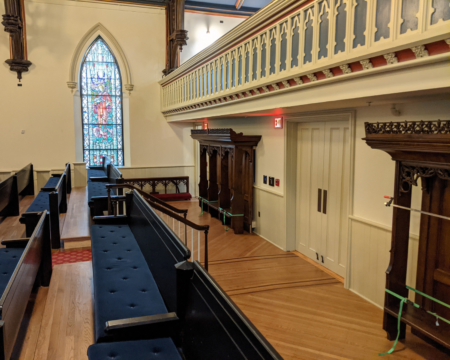The photograph captures the interior of a quaint church, offering a detailed view from the entrance. The church's design emphasizes a palette of beige and light yellow hues that bathe the walls, giving the space a warm and inviting ambiance. The focal point of the background is a stunning arched stained glass window that casts colorful reflections across the room. The entrance door, a deeper shade of tan beige, invites visitors into this sacred space.

Upon entering, you traverse a few steps with dark brown wooden railings adorned with matching beige spindles. The flooring is a polished medium brown wood that gleams under the light. The spacious single-story structure features a choir loft on the right, marked by yellow banister strips with red accents and intricate gray glass decorations below, all supported by light yellow paneling.

To the left of the double entry doors, which flaunt flat metal handles, stands a dark wooden cabinet. Another cabinet, roped off with green and yellow ribbon, is situated to the right of the doors. The long, dark cherry wood pews, aligned in neat rows, are equipped with black cushions for seating, while their backs remain bare wood. The pews' arrangement creates a harmonious contrast with the bright blue and dark wood elements of the altar and surrounding areas.

The image captures the essence of a serene morning inside the church, highlighted by various architectural features such as black chairs notable against the light brown floor, and light fixtures hinting at a second level. The entire scene is tied together with a red carpet featuring delicate yellow designs that lead towards the altar, providing a central path through this peaceful sanctuary.